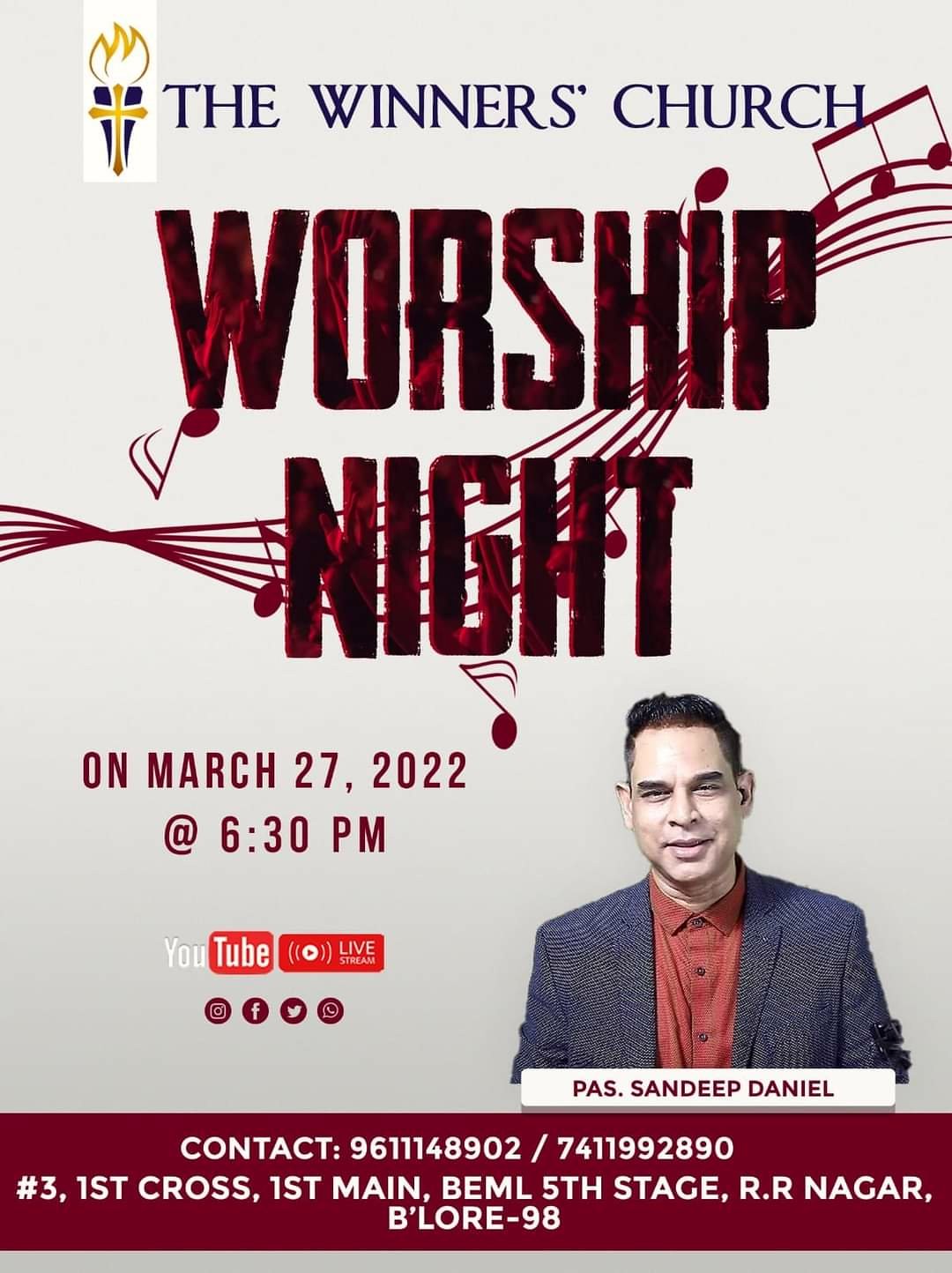The poster, set against a light grayish background, announces an event for The Winner's Church. At the top left corner is an emblem of a torch, with a cross forming the handle and topped with a yellow flame. Centrally placed at the top is the church's name, "The Winner's Church," followed by the event title, "Worship Night," boldly displayed in creative red and black fonts, with a treble clef and assorted musical notes winding through the text in a striking red color. 

The event details follow beneath: Scheduled for March 27th, 2022, at 6:30 PM. Indicated below are logos for YouTube live stream and social media icons for Instagram, Facebook, Twitter, and WhatsApp, indicating the event's online presence. 

On the right side of the poster is a photograph of a man identified as Pastor Sandeep Daniel. He is depicted in a red shirt buttoned to the neck, over which he wears a black or dark blue blazer. He appears clean-shaven with short black hair.

The bottom of the poster features a horizontal maroon strip, which includes contact information: 961-114-48902 or 741-199-2890, and a location: #3 First Cross, BML 5th Stage, RR Nagar, Bangalore 98. This detailed layout serves as a captivating and informative announcement for the upcoming worship night.